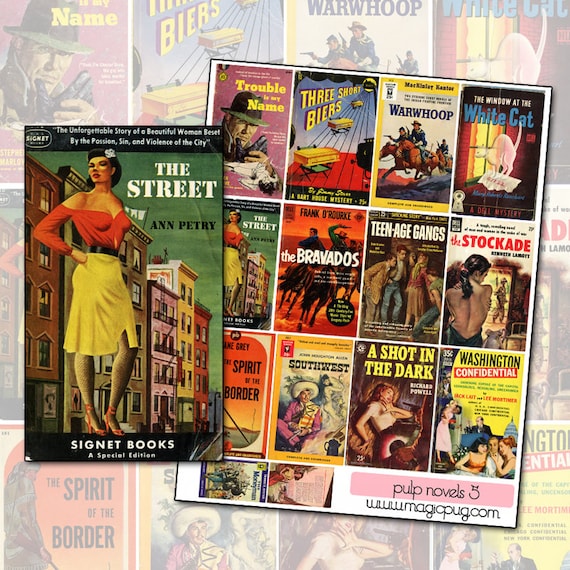This image displays a collection of vintage pulp novel covers arranged in a grid-like format with several rows. Emphasized prominently is the cover for "The Street" by Ann Petry, featuring a woman in a tight, shoulderless red top, black belt, knee-length yellow skirt, fishnet stockings, and red, thin-strapped heels. She has dark, shoulder-length hair adorned with a flower and is looking over her shoulder at a backdrop of four or five-story buildings. The ensemble includes titles like "Trouble is My Name," which sports a pink cover with a man in a fedora and trench coat; "Three Short Beers," depicted with elements including coffins and horizontal lines; and "War Whoop," showing men with guns riding horses. Other titles include "The Window at the White Cat" featuring a scary Siamese cat, "The Bravados" with cowboys, "Teenage Gangs" depicting a group of kids, "The Stockade" with a bareback figure, "Southwest," "A Shot in the Dark" with a distressed woman, and "Washington Confidential," hinting at political scandals in Washington D.C. The background subtly fades, with some titles slightly tilted to the right, emphasizing the nostalgic and eclectic mix of pulp fiction. At the top, the line "Pulp Novels 3" is visible alongside the URL www.magicpug.com.